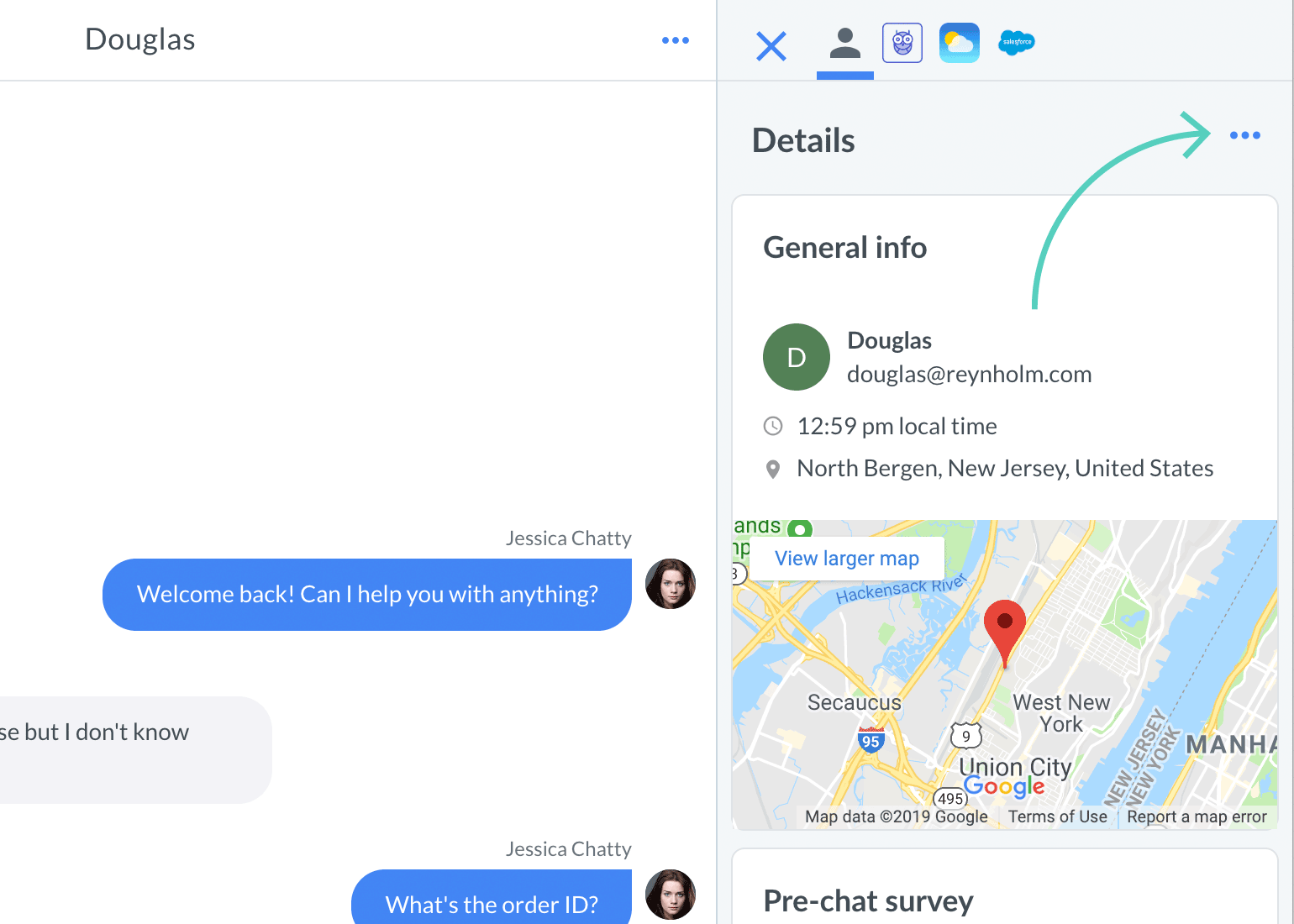The image consists of two detailed screenshots. The screenshot on the left shows a white background with the name "Douglas" at the top, indicating it is a part of a text conversation. The dialogue reads, "Jessica Chatty, welcome back. Can I help you with anything?" Douglas's reply is visible but mostly cut off, with only the phrase "but I don't know" readable. Jessica Chatty responds with a query, "What's the order ID?"

On the right side, there is a section titled "Details" containing general information about Douglas, specifically his email: Douglas@reynholm.com. A curved green arrow on the screenshot points upwards to the right, indicating a prompt to click on three horizontal circles. The timestamp reads "12:59 p.m. local time," and the location is North Bergen, New Jersey, United States. Below this, there is a screenshot of a Google Map with a pin marking a specific location. The map includes labels such as "pre-chat survey" and notes like "map data, copyright 2019, Google, terms of use, report a map error." Both screenshots are devoid of any images of animals, plants, flowers, trees, or buildings.